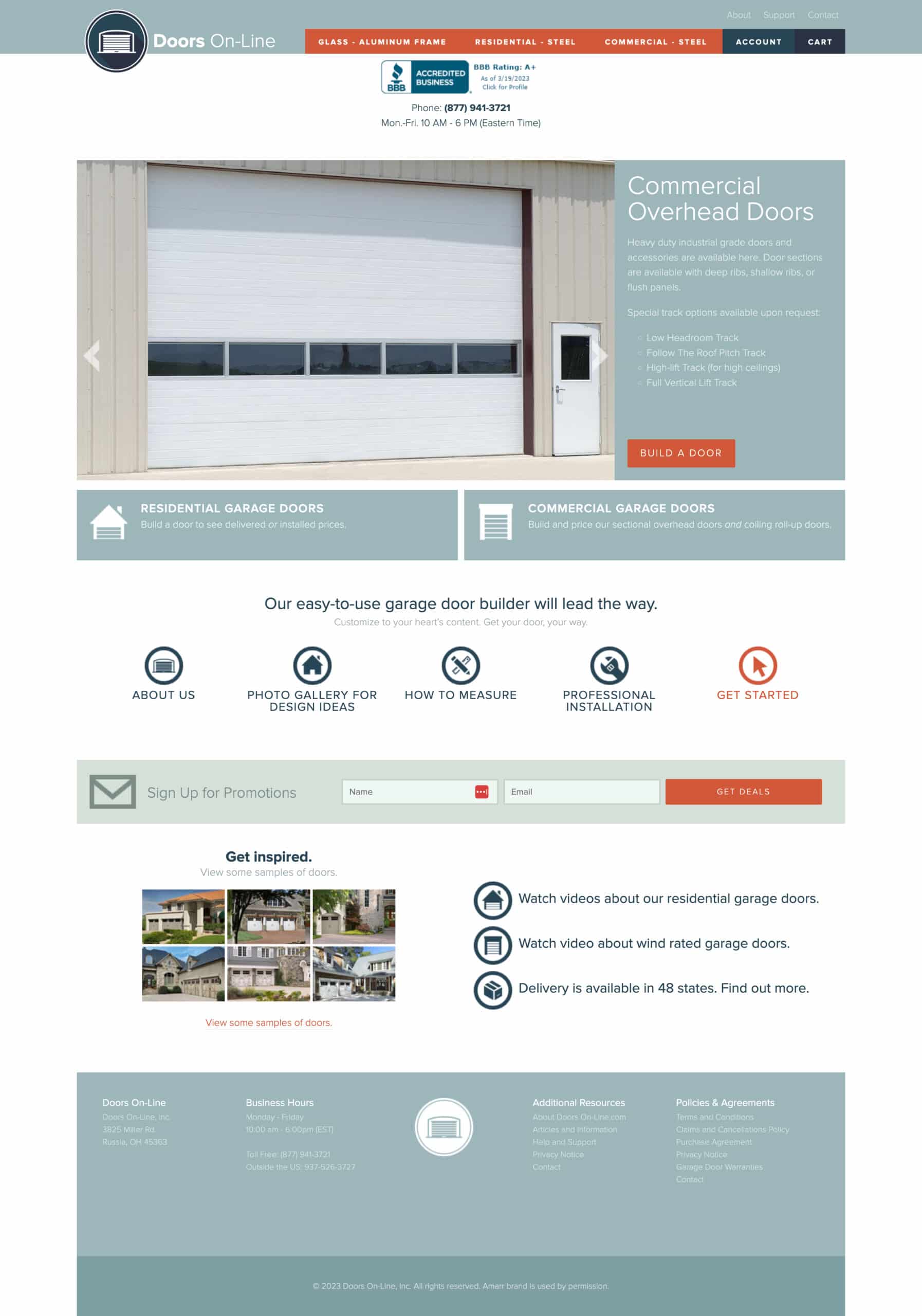This image is a screenshot of the 'Doors Online' website. The focus appears to be on the header of the site, highlighting its various elements. At the top left of the screenshot, there is the 'Doors Online' logo, featuring a stylized white garage door emblem against a dark green background. To the right of the logo, the site name is displayed with 'Doors' in bold white text, and 'Online' in regular white text with a hyphen connecting 'On-' and 'line'.

Moving towards the top right section, there is a series of navigation tabs labeled from left to right: 'Glass', 'Aluminum Frame', 'Residential Steel', 'Commercial Steel', 'Account', and 'Cart'. Each tab is distinctly colored, making it difficult to determine the active page; 'Account' is highlighted in green, 'Cart' in black, and 'Aluminum Frame' and 'Residential and Commercial Steel' are in orange.

Further to the right, there are three additional buttons: 'About', 'Support', and 'Contact'. Centrally at the top of the page, the company's phone number and business hours, which are 10 a.m. to either 8 p.m. or 6 p.m., are displayed. Lastly, some information regarding their commercial overhead doors can be seen in the middle section of the screenshot.